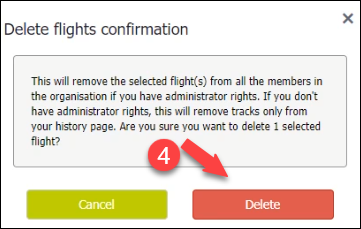The image appears to be a screenshot from a digital interface, such as a website, webpage, or an application. The image is in a smaller horizontal format and is surrounded by a thin black border. The primary background inside the border is a stark white, typical of a computer screen's native color.

At the top left corner of the image, there is text in a muted black font that reads "Delete Flights Confirmation." Opposite this text on the top right corner, there is a clickable 'X' button, commonly used for closing the window.

Beneath this header, there is a horizontally oriented, gray rectangular box with slightly rounded corners. The box contains the following text: "This will remove the selected flights from all the members in this organization if you have administrator rights. If you don't have administrator rights, this will remove tracks only from your history page. Are you sure you want to delete one selected flight?"

Additionally, a red circle featuring the number '4' is displayed with an arrow pointing towards a red 'Delete' button below the grey text box. Next to the red 'Delete' button, there is also a green 'Cancel' button that users can click on to abort the deletion process.